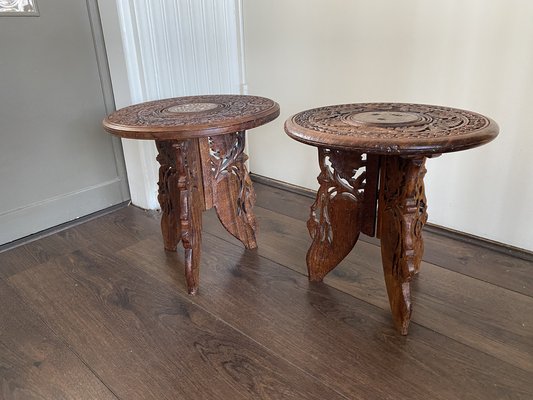The image showcases two identical, antique-style side tables positioned on a dark walnut-colored hardwood floor. Both tables feature round tops with detailed circular carvings or inlays at the center. Each tabletop is supported by three wide, flat legs that appear to be intricately shaped from planks of wood, almost suggesting that they could fold up. The background comprises a mix of a light gray wall and what seems to be a partially visible white curtain or blinds toward the upper left. The setting includes an off-white wall section near the center, possibly indicating an adjacent door or another wall, adding subtle depth to the scene. The photo angle restricts the visibility of the finer details on the top of the tables.